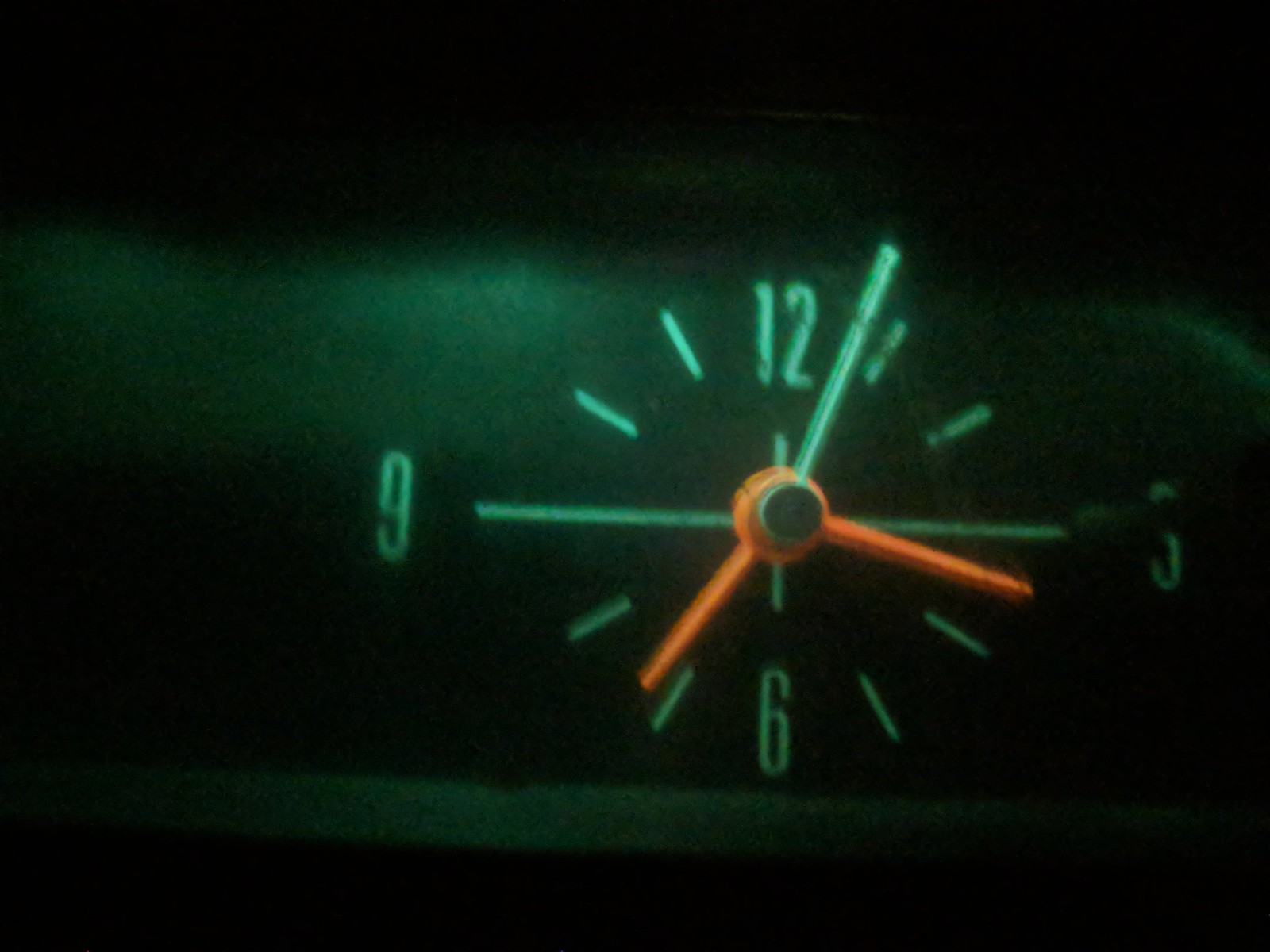A close-up image depicts a vintage dashboard clock, reminiscent of those found in classic automobiles. The clock face is predominantly black, providing a stark contrast to its details. In this monochromatic setting, the numbers on the clock are distinctly marked: 12 at the top, followed by two short lines before the 3, then continuing with three, two short lines before the 6, another two short lines, the 9, and finally two short lines completing the circle back to 12. The clock hands, exhibiting a warm, orangish hue, indicate the time as approximately 7:17. Adding an additional layer of character, a subtle green tone permeates the entire image, casting a nostalgic, almost cinematic ambiance.